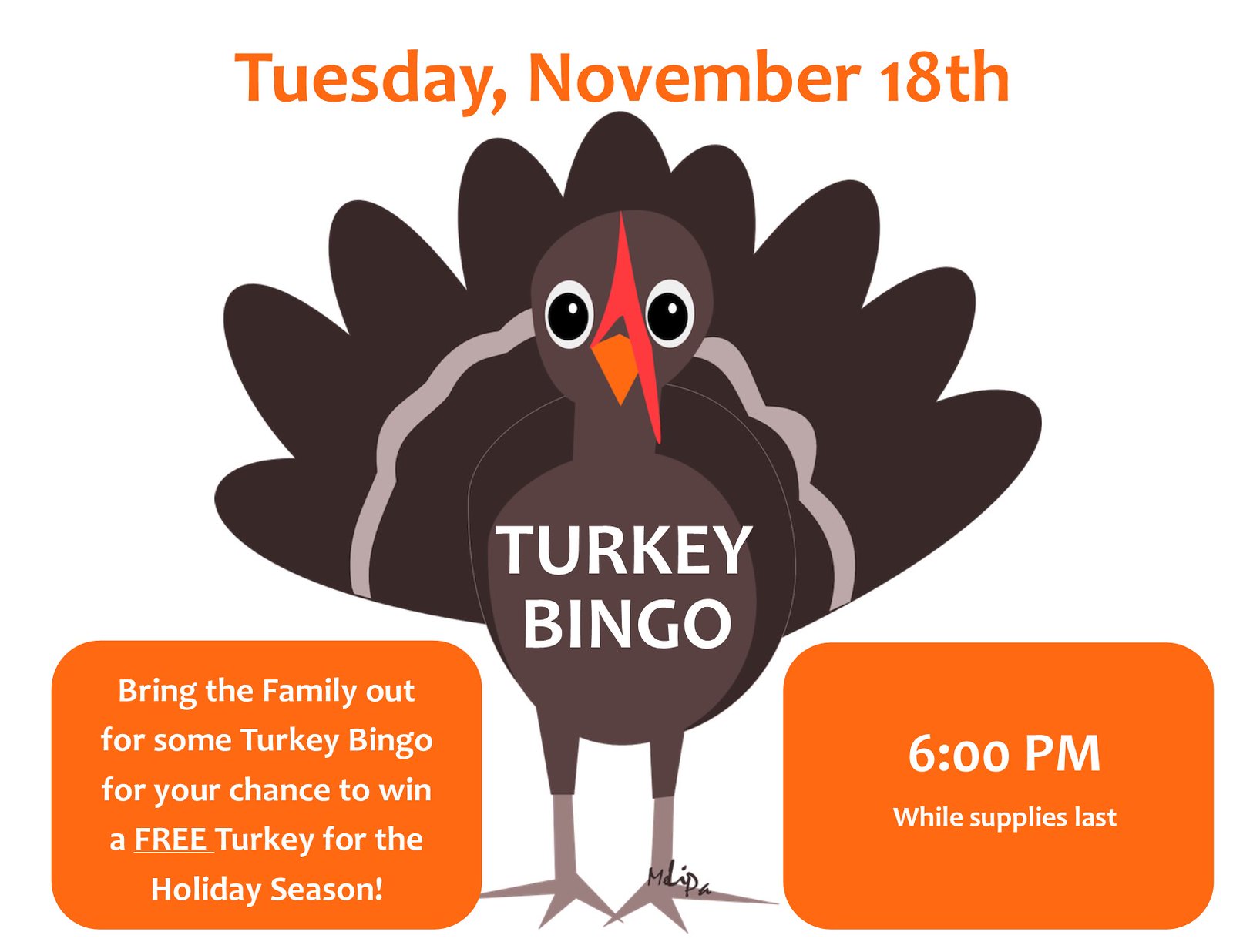The image displays a digital advertisement prominently featuring a cartoonish turkey at its center. The turkey, depicted in varying shades of gray, has distinct black eyes, an orange beak, and a red wattle. At the top of the image, in vibrant orange and red letters, the date "Tuesday, November 18th" is displayed. On the turkey's chest, the text "Turkey Bingo" is written in bold white letters. Flanking the turkey are two gold rectangular boxes with rounded corners: the box on the left invites families to "bring the family out for some turkey bingo for your chance to win a free turkey for the holiday season!" while the box on the right states the event timing as "6pm while supplies last." The advertisement lacks a background and border, focusing attention on the turkey and the event details.